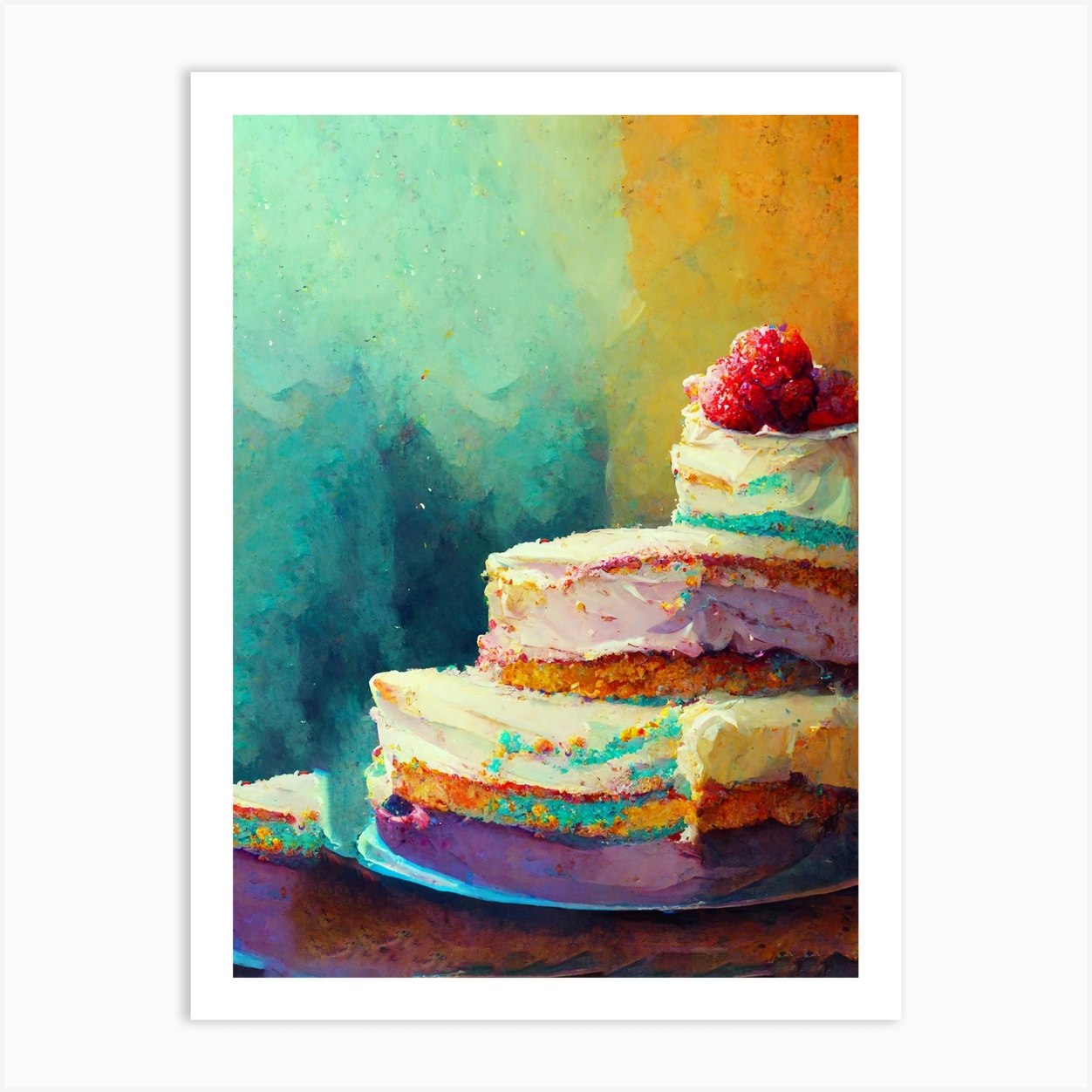The painting depicts a vibrant three-tiered cake with a striking watercolor backdrop. The cake, styled like a naked cake, features three distinct layers: the bottom layer is thick with white buttercream frosting and cake crumbs, the middle layer is taller with a purplish tinge to the frosting, and the top layer is the thickest, smallest, and least wide, adorned with clumps of red berries. The background transitions from a light greenish-blue at the top, merging into deeper blues on the left and mustard yellow on the right, creating a vivid and colorful scene. Detailed gold and purple bands embellish the lower part of the image, adding to the vibrancy. The painting itself is outlined or framed in white, enhancing the bright and clear presentation with ample natural lighting.